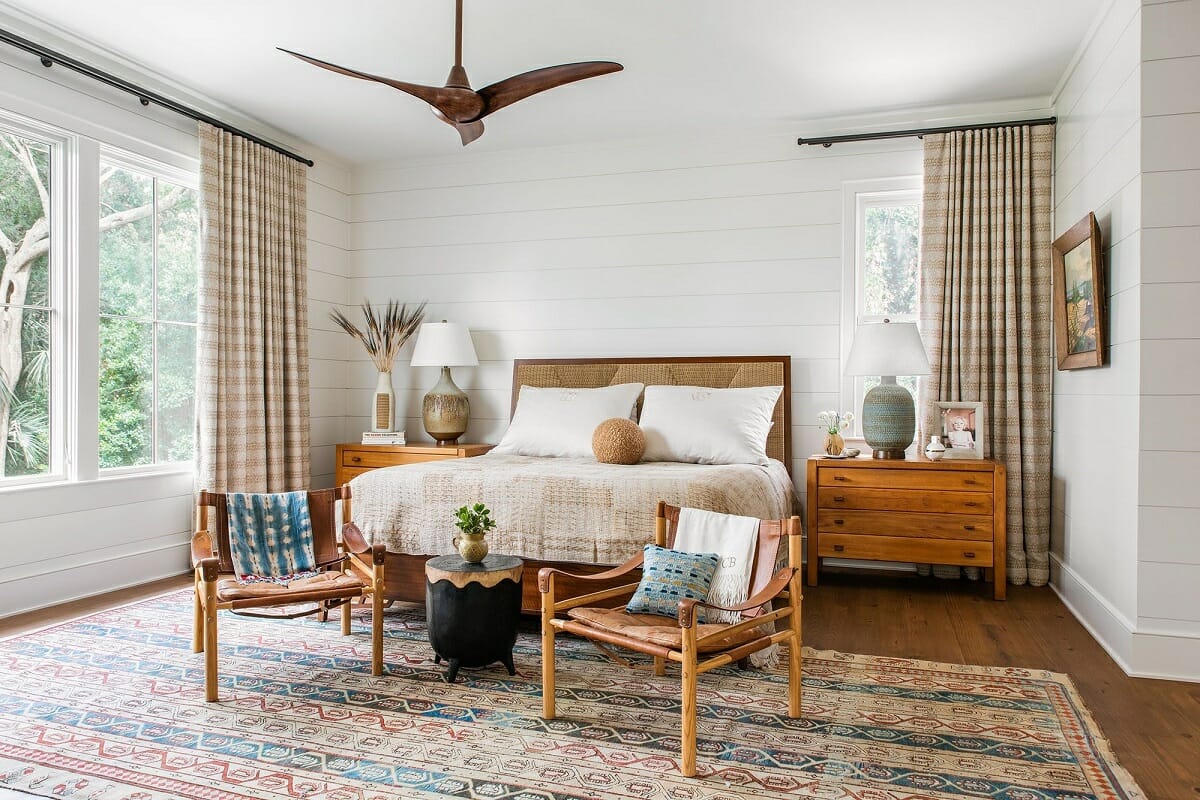The horizontally aligned rectangular picture captures a serene bedroom interior. The walls are adorned with horizontal white wood planks, contributing to a calm, natural vibe. To the left, there are two large rectangular windows framed with white wood and adorned with plaid curtains in brown and beige, pulled back to reveal green trees outside. On the right wall, there is another window with matching curtains. 

Central to the room is a neatly made bed featuring beige sheets and a headboard with a dark brown wood frame. It is accessorized with two white pillows and a distinctive round brown pillow placed between them. Flanking the bed are two medium-toned wooden nightstands, supporting lamps, picture frames, and small flower pots.

In front of the bed, two brown wooden chairs are positioned with a small round table between them, which holds a potted plant. A patterned area rug with hues of blue, brown, and red featuring curved lines rests beneath the furniture on dark brown wood tile flooring, adding warmth to the space. The room also includes a minimalistic white ceiling fan with wooden blades and a painting hanging on the right wall, enhancing the room's tranquil and cohesive decor.